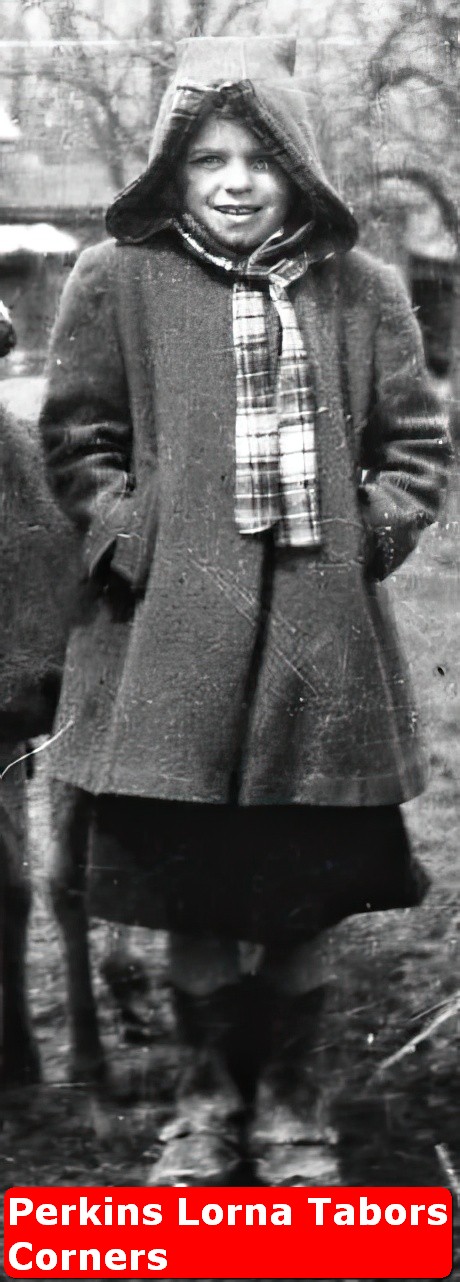The black and white image depicts a smiling young person, possibly a historical figure, looking directly into the camera with their top teeth visible. The person, whose androgynous appearance makes it hard to determine their gender, is dressed in winter clothing—including a long jacket with a hood, a checker-patterned scarf, and cowboy boots. Their hands are tucked into their pockets, suggesting a cold environment, possibly with snow as hinted by the background featuring what appears to be a farm setting. The photograph shows signs of aging, with noticeable damage such as folds or scuffs at the top. At the bottom, against a red background, white text reads "Perkins, Lorna, Tabers, Corners," possibly indicating the individual's name or a notable location related to them.